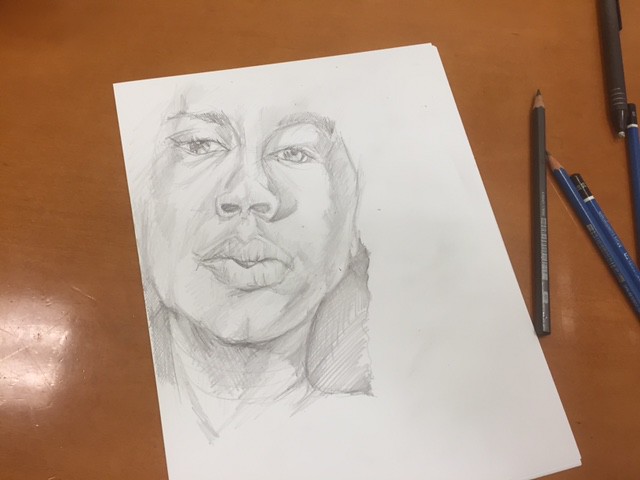In this image, a slightly slanted white piece of paper rests on a light brown desk. The paper features a detailed sketch of a face positioned in the top left corner. The artist has intricately drawn the eyebrows, eyes, and nose, with visible shadowing to enhance the nose, while the lips appear slightly larger than usual. The sketch also includes the beginnings of a background and the outline of the person’s neck.

To the right of the paper lie three pencils and a pen. The pencils include a gray one, a blue one, and another blue one which is positioned such that only its end is visible. Additionally, there is a gray pen-like object placed slightly above the pencils. The assortment of drawing tools suggests active use in the creation of the detailed facial sketch.